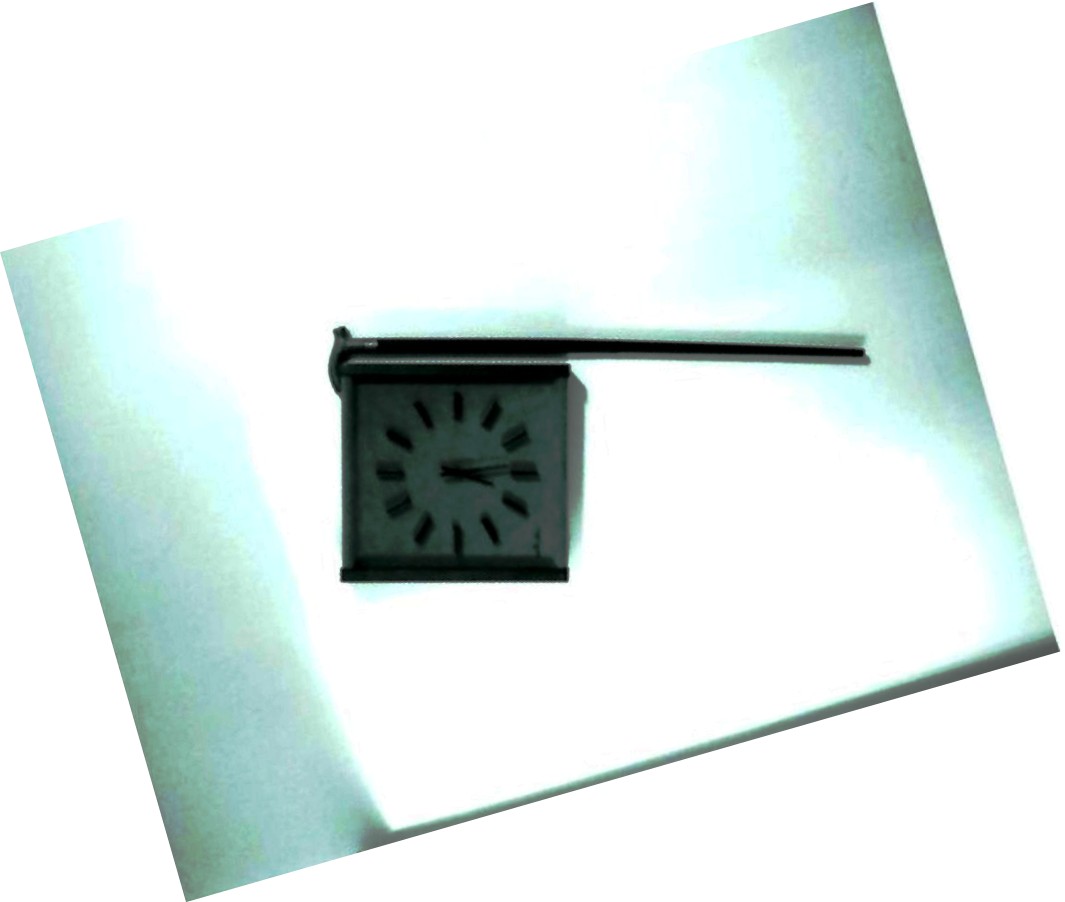This color photograph, slightly tilted and set against a white backdrop, features unique lighting that creates a subtle blue halo around its edges. The image captures a square, white metal clock, distinguished by its minimalist design where each hour is marked by a simple black line. The time displayed is 4:14. The clock, accentuated by black borders at its top and bottom, hangs from a sleek metal bar, predominantly black but with a touch of silver on the left side. The overall visual effect is striking, with the clock's monochrome palette contrasting sharply against the unusual lighting and the stark white background.